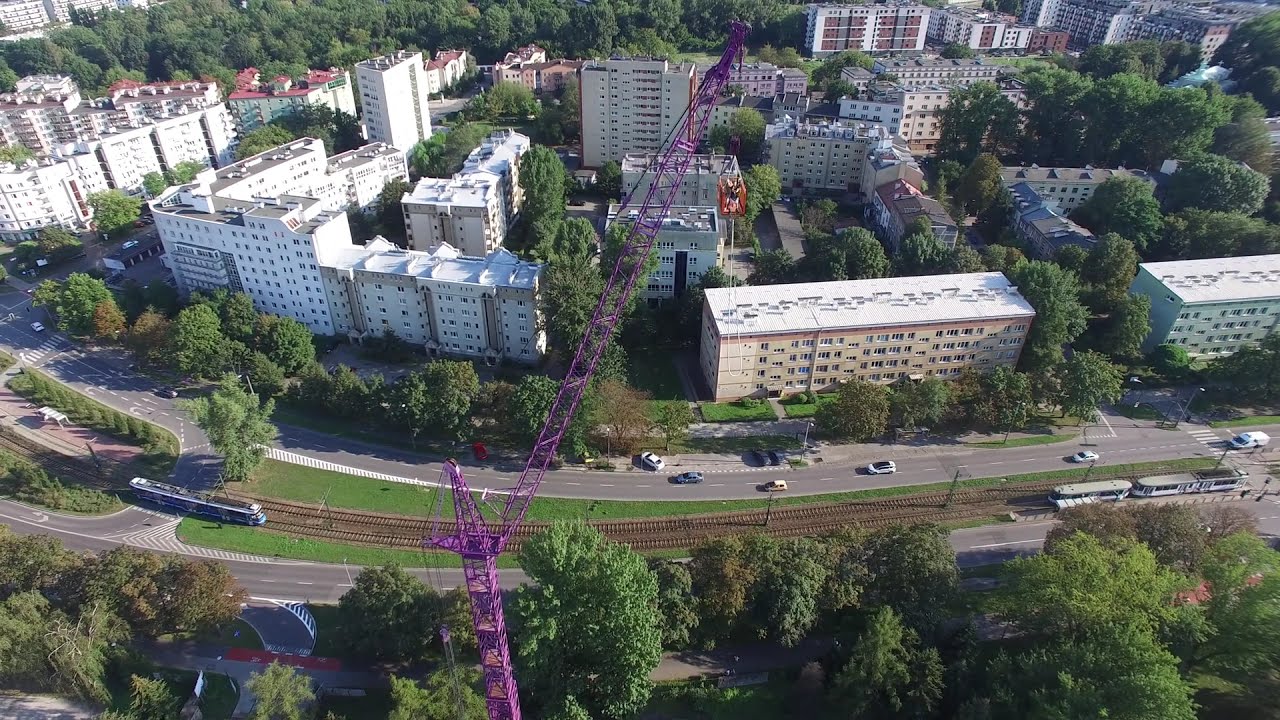An overhead, aerial photograph showcases a bustling section of a city bathed in bright daylight. Dominating the forefront is a prominent purple construction crane, its arm extending and holding what seems to be a cage, though it’s unclear if it’s occupied. Below the crane is a two-lane road running horizontally across the image, populated by six or seven cars. To the right of this road lie train tracks, hosting two trains—one moving and one stationary—with possible train platform buildings adjacent. This two-lane road appears to separate two zones; multiple five-story buildings, predominantly white with some light brown structures, occupy the background. Trees are interspersed among the buildings and around the area, their lush green foliage adding vibrancy to the urban landscape. The tops of the buildings also reveal some patches of red. There’s no visible sky or people, just the man-made and natural elements of the city captured from a high vantage point.